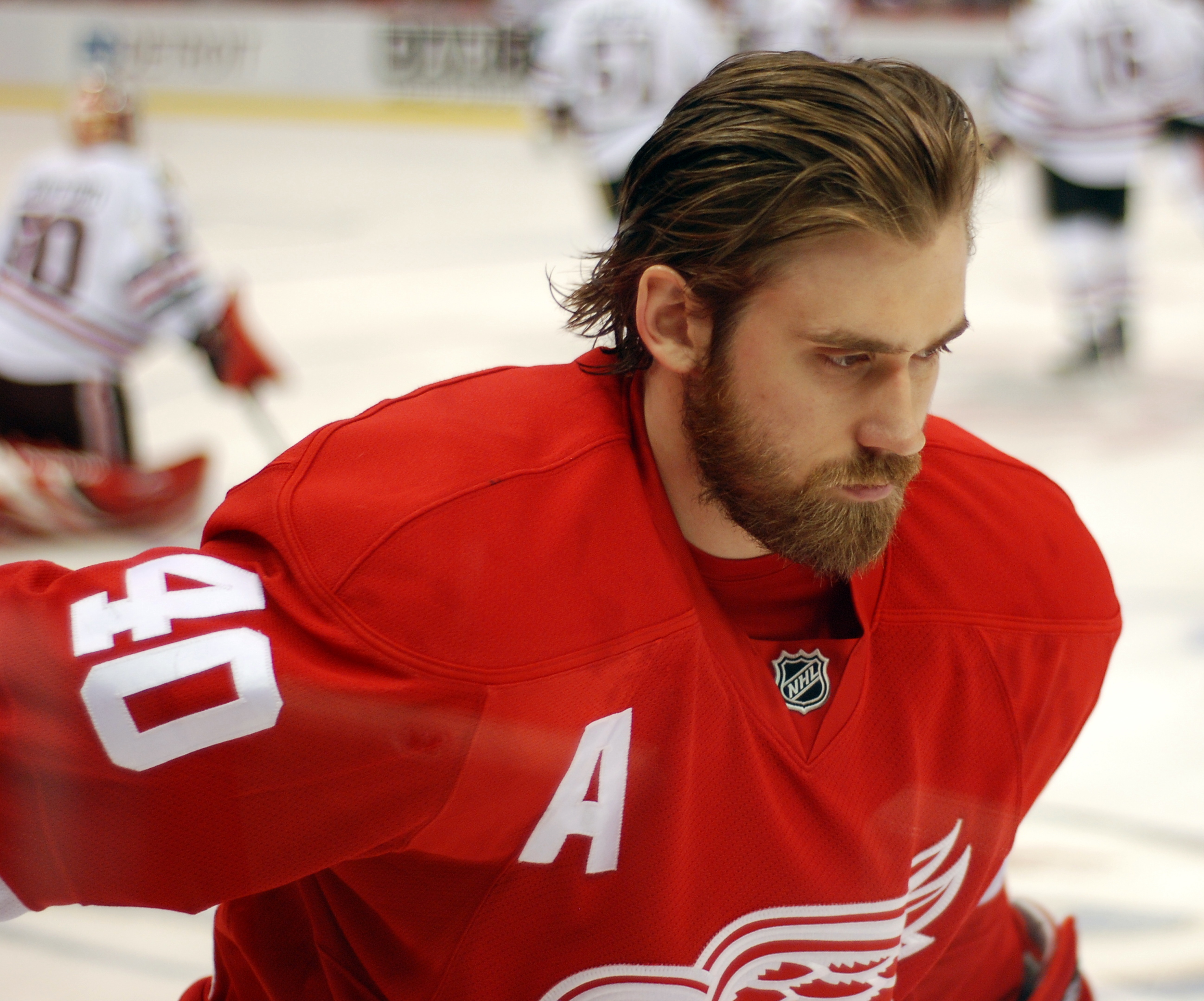This image depicts a professional NHL player from the Detroit Red Wings, captured in a solemn moment on the hockey rink. The player, a white male in his 30s, stands out with his neatly slicked-back short brown hair, full brown beard, and moustache. He is wearing a vibrant red jersey prominently featuring the number 40 on the sleeve and a bold white "A" on the chest, signifying his status as an alternate captain. Just beneath the "A," a subtle white design hints at the team's iconic logo. The NHL logo, displayed in white on a black background, is positioned at the top center of the jersey. The player gazes downward, seemingly lost in thought. In the out-of-focus background, blurry figures in jerseys of white, black, and red colors populate the hockey rink, highlighting the primary subject's sharp clarity in this portrait shot.